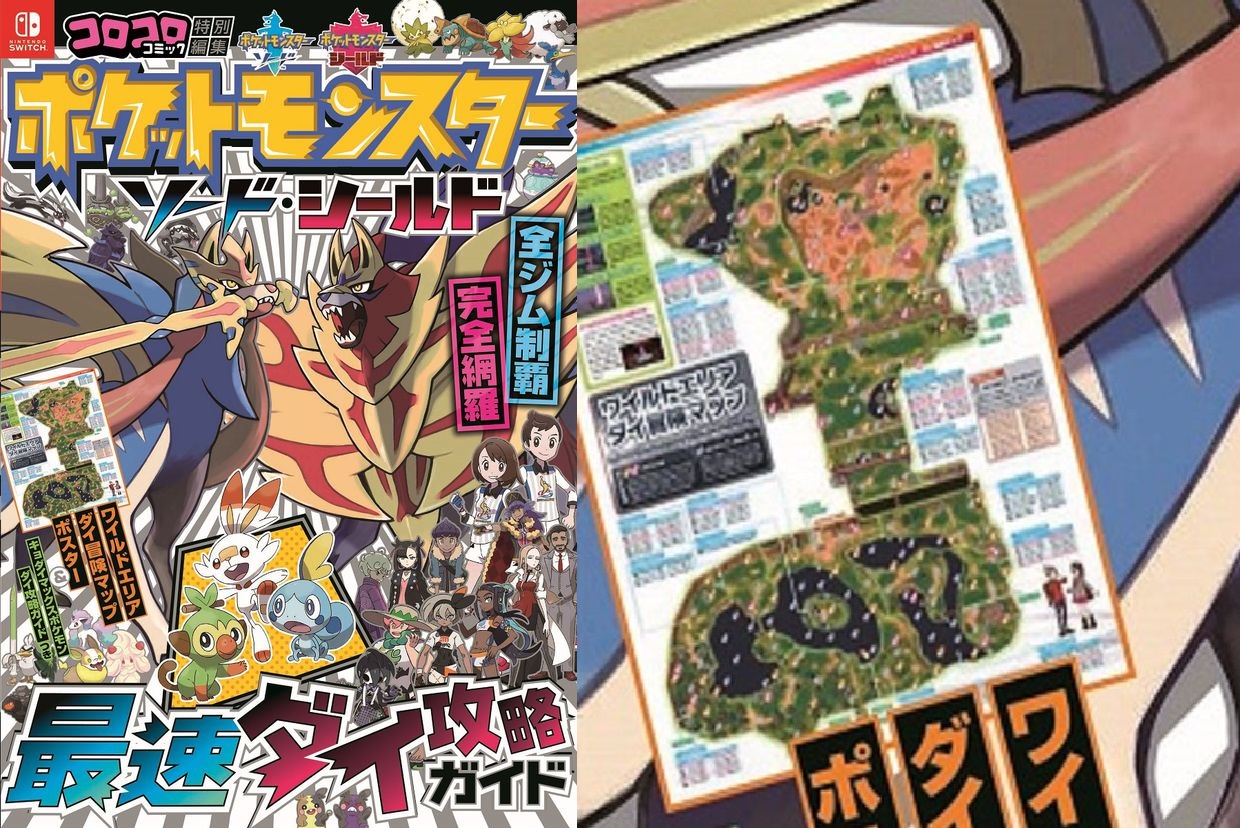Promotional Image for Pokémon Nintendo Switch Game, Featuring a Bonus Map

This promotional image showcases an upcoming Pokémon game (or set of games) for the Nintendo Switch, with all text displayed in Japanese. Prominently featured on the cover are several Pokémon characters along with a variety of human figures presumed to be Pokémon trainers. 

In the upper left corner, the familiar Nintendo Switch logo is visible, with the iconic two Joy-Cons depicted in white against a red background, and "Nintendo Switch" written below. To the right of this main image, there appears to be an inset featuring a detailed section of a map. This map, seemingly included as part of the game package, is illustrated with notations and various cartographic elements. 

The inclusion of this zoomed-in map section suggests that purchasers of the game will receive the map as a bonus item. The photograph aims to highlight this special inclusion, giving potential buyers a preview of the detailed map that accompanies the game.